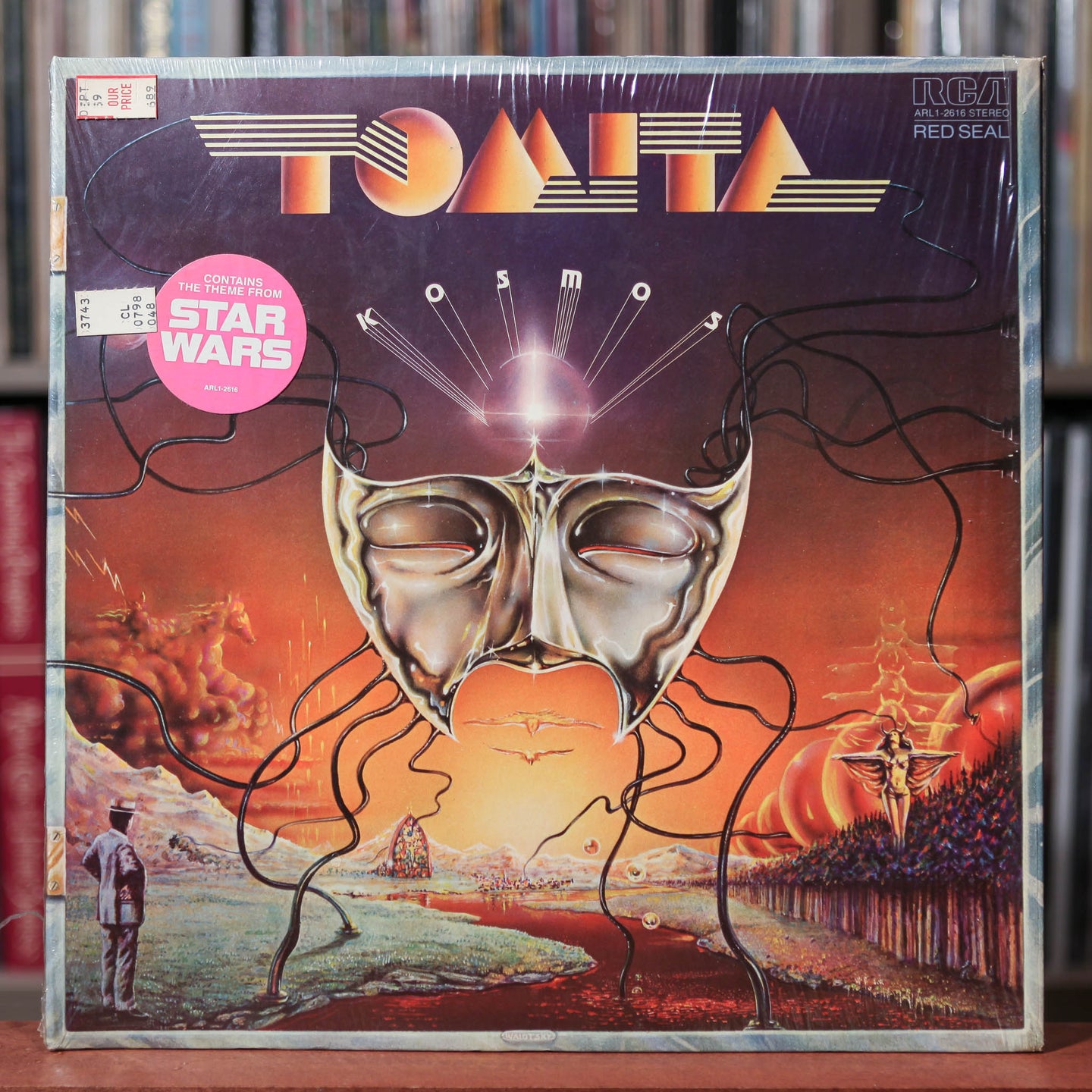The image is of a vintage album cover, likely from the 1970s or 1980s, propped up on a slightly red-colored table with out-of-focus shelves stocked with other albums in the background. The cover prominently features the title "Cosmos" in white letters, positioned in an arc below geometric letters at the top that seemingly spell "Tomita." The album, associated with an exotic modern art theme and advertised as containing the theme from Star Wars, bears a pink sticker and other serial-numbered labels, along with an RCA logo in the top right corner.

Dominating the album cover's design is an opera-style gold mask with eyes closed, from which various vines or tentacle-like limbs extend across an orange-gold background. Below the mask, there is a surreal scene with a small creek at the bottom left, where a man in a hat and suit stands on green ground, looking away. The right side showcases a grove of reddish-brown trees and a woman in a bikini with wings, appearing to ascend. The overall palette is a vivid mix of oranges, purples, reds, and blacks, creating a striking and eclectic piece of modern art.